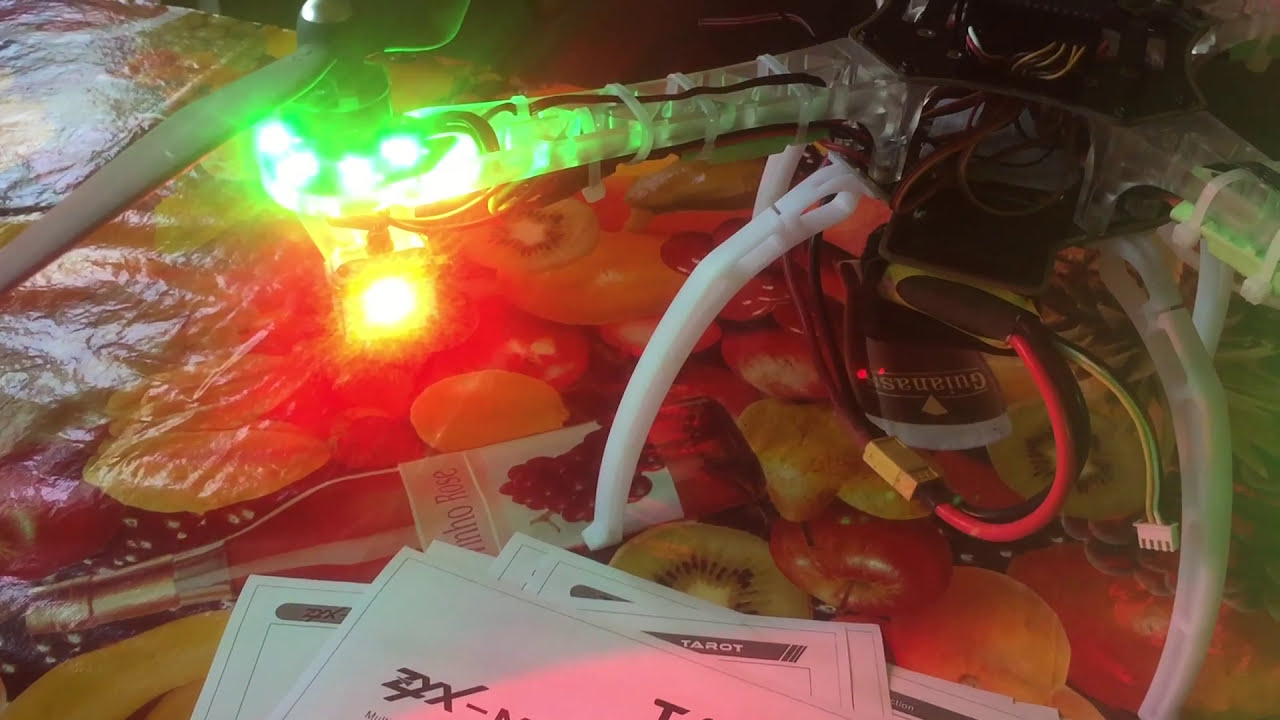The image features a deconstructed or partially assembled drone situated on a colorful tablecloth adorned with images of fruit and alcohol. The drone, positioned in the top right of the image, displays visible exposed wires and LEDs, with some parts of its plastic casing missing, suggesting it is in the process of being built or modified. Notable features include a propeller in the top left-hand corner and several zip ties securing components along one of the drone's arms. 

On the surface around the drone, various objects are strewn about. To the right of the drone, there appears to be a headset with earphones and a head-mounted camera. In the background to the left, a green stick-like object with glowing lights is visible. Several identical placards lay haphazardly at the forefront, some bearing inscriptions like "tarot" and "Z-Y-X," with parts of the latter obscured. Additionally, a bottle resembling a pink wine bottle lies on its side nearby, though it is unclear if it is a physical object or part of the tablecloth design. Scattered among these items, there are circular objects, one of which looks like a slice of fruit with seeds in the center. The scene is chaotic, with elements of illumination giving the impression of light filtering through or reflecting off plastic, creating an interplay of green, white, and orangish-red hues.